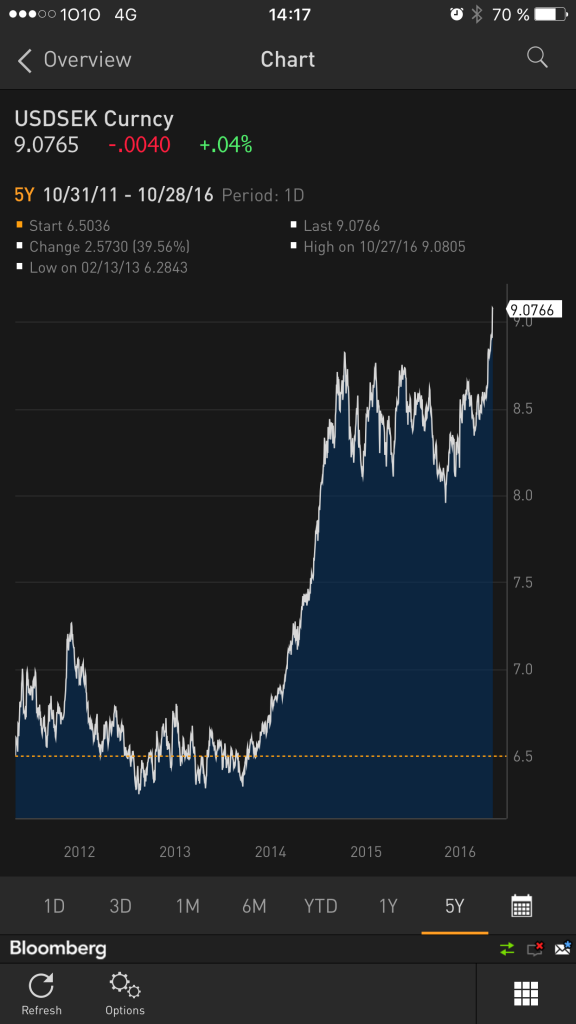This image is a detailed screenshot taken from a smartphone displaying a financial chart, likely from a stock-tracking or currency exchange app. In the top left corner, the phone shows signal strength with three out of five bars and indicates a 4G connection. The current time is 14:17, and icons for an active alarm, Bluetooth connectivity, and a 70% battery life are visible.

The top of the app interface features navigational elements including a left-pointing arrow labeled "Overview," next to which there is a "Chart" section that is highlighted, and a magnifying glass icon for search.

Below this navigation, the details for the USD/SEK currency pair are displayed. The current rate is 9.065, having decreased by 0.0040 or -0.04% in the latest session. The data spans five years (5Y), with the rate oscillating between a high of 10.2716 and a low of 6.2843 within this period.

Highlighted metrics include:
- Period: 1 Day (1D)
- Start: 6.5036
- Change: 2.5730 or 39.56%
- Last rate: 9.0766
- High recorded on the chart: 9.0805

Beneath this data is a graph showing the historical performance of the currency pair. It starts low and exhibits a sharp spike in the middle. A white label on the graph marks the point 9.0766. The timeline at the bottom ranges from 2012 to 2016, with options to view different periods including 1D, 3D, 1M, 6M, YTD, 1Y, and 5Y, the latter of which is currently selected.

At the bottom of the screen, there are buttons for "Bloomberg," "Refresh," and "Options," indicating that the interface likely belongs to a Bloomberg financial tool.